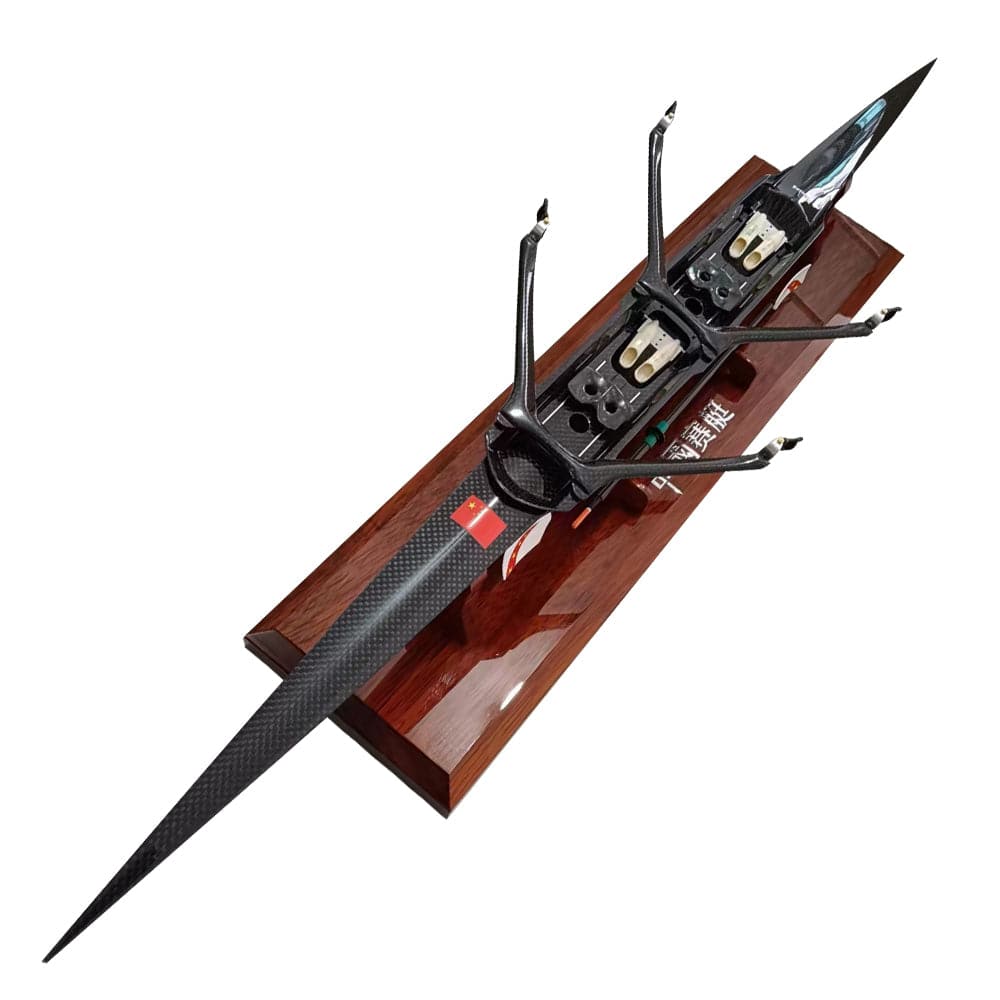This photograph captures a detailed bird's eye view of a sleek black racing boat model, meticulously displayed on a dark brown stained wooden base. The base, designed in a diagonal layout, prominently features white Chinese characters in its center, enhancing its cultural distinction. The long, slender boat, resembling a kayak, extends beyond the rectangular stand with a pointed prow. Distinctive markers include two pairs of white shoes inside the boat, indicating seating positions for rowers, further accentuated by a clear cover at the front. A small red box, potentially housing other model components, is situated behind the seating area. The model is adorned with a painted Chinese flag near the rear and a flag on the right front side, emphasizing its national affiliation. On either side of the boat, metal arms suggest the presence of oars, underscoring its design as a racing vessel. The overall display, despite the lack of a descriptive heading, vividly illustrates a sophisticated, culturally enriched rowing boat model.